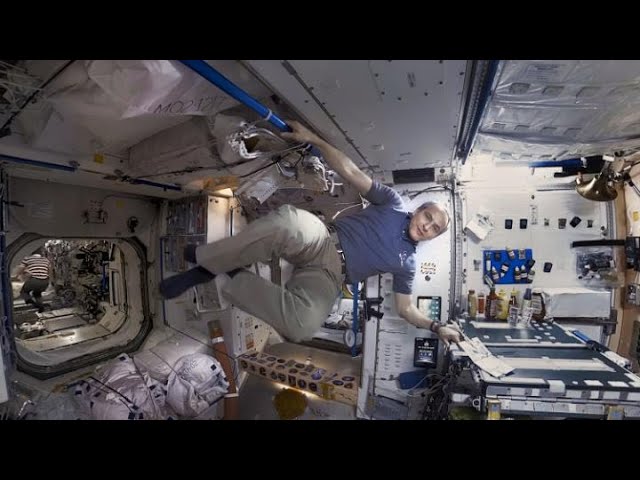In this detailed full-color photograph taken outdoors using artificial light, we are given a glimpse inside the International Space Station. The square image is framed by a black border on the top and bottom, though the photo itself is vertically rectangular. At the center, a Caucasian man with possibly gray or white hair, which might just be a trick of the light, floats in mid-air, secured by his right hand gripping a blue pipe. He is dressed in a blue polo shirt, tan khaki pants, and dark-colored socks, likely black. His left hand grazes a paper on a black-surfaced desk. The area appears somewhat cramped, contributing to the sense of a bustling yet confined workspace in zero gravity.

To the left, another astronaut in a white and red horizontally-striped shirt and brown pants can be seen navigating through the space station. The interior features predominantly white walls and ceiling, contrasted by a gray floor. Various items, including bottles of sauces, suggest the everyday routines these astronauts maintain. Through an opening at the man's feet, another room of the spacecraft is visible, enhancing the immersive feel of this extraordinary scene.